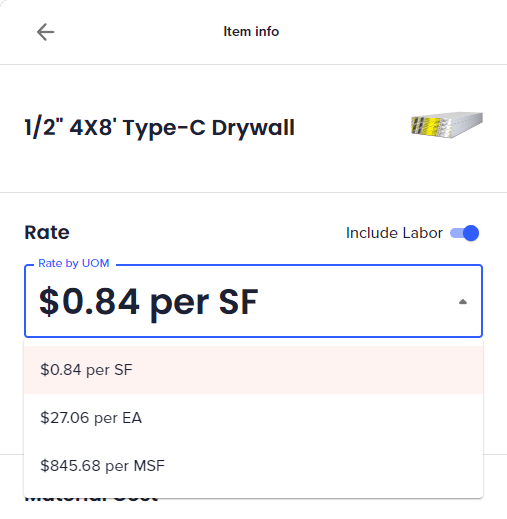The image displays a user interface related to drywall purchase options. It features a 'Back' arrow and the text "Item Info" in black at the top. Below, it presents details about the drywall, labeled as "1/2" four times eight, Type C, Drywall." The drywall appears to be silver with a yellow center.

Further down, the interface showcases pricing information under the heading "Rate" and "Rate by UOM," highlighted by a blue box. An active "Include Labor" filter affects the pricing. Three pricing options are listed in a chart, allowing for easy selection between different measurements:

1. $0.84 per square foot (selected).
2. $27.06 per EA.
3. $845.68 per MSF.

The text is primarily black on a white background, accompanied by a few images and an interactive blue button.